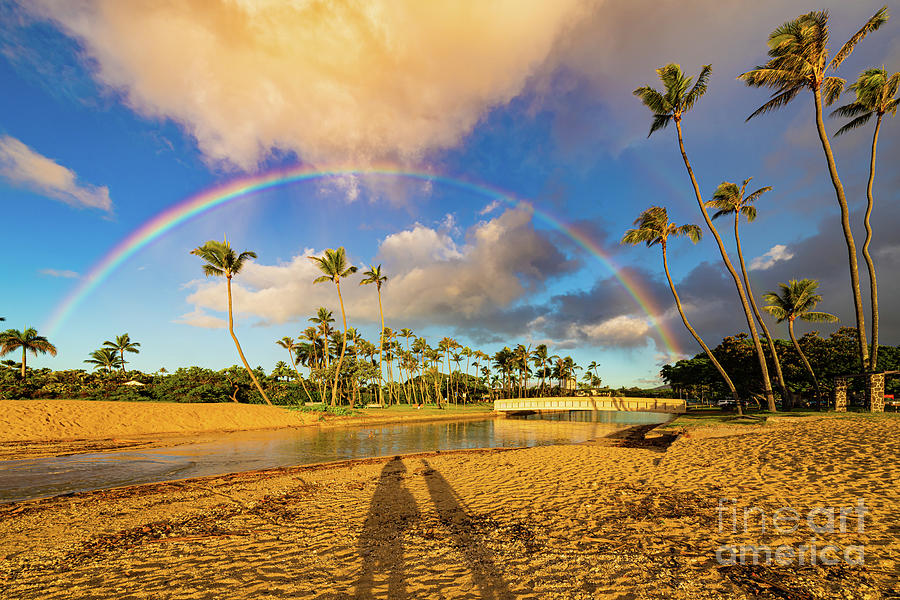The image portrays a vibrant tropical scene characterized by deep blue skies and enhanced colors. Dominating the sky is a full, arching rainbow that extends from the left middle part of the image and arches toward the right, ending at a bridge over a stream or river running through the middle of the picture. Puffy white and golden clouds accentuate the rainbow's vivid hues. Below the rainbow, a variety of palm trees, including some with irregularly shaped trunks, populate the landscape, with some standing taller and closer in the foreground and others smaller in the background. The foreground features golden-yellow sand marked by numerous depressions from footsteps, and the shadows of two people—the person taking the photograph and possibly a tall thin object, such as a camera tripod. The sandy beach lines both sides of the stream, highlighting a scene that combines natural beauty with human presence.